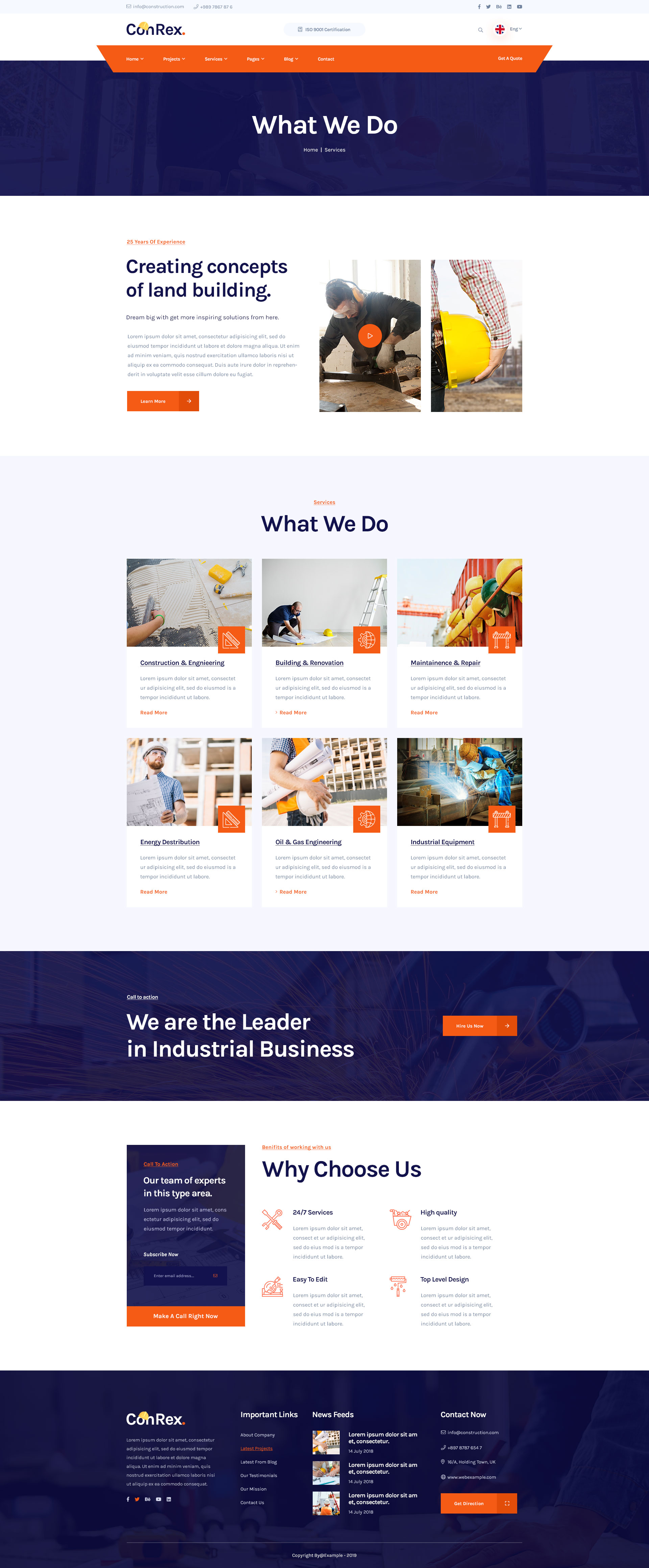This image is a portrait-mode screenshot of the Conrex website, showcasing various sections of its user interface. In the upper-left corner, "CONREX" appears in white against the background. The upper-right corner features what looks like a British flag. Below this is an orange navigation bar with tab headers that are too small to read.

The next section features a large blue background with the text "What we do" in very small font, followed by even smaller text stating "Home services." This area appears largely empty, with excessive unused space.

Following the blue section, the text "Creating concepts of land building" appears, with a video thumbnail to the right showing a construction scene. The video can be played by clicking the orange button with a play icon. Next to this image is another, depicting a person holding a yellow helmet. Below the "Creating concepts of land building" text is a paragraph that is too small to read, accompanied by an orange button, likely labeled "Learn More."

The next part of the screenshot features a "What we do" section, presenting images and brief descriptions, which seem to be blog entries. This is followed by another extensive blue section with the text "We are the leader in industrial business" and a very small, unreadable orange button on the right.

The subsequent segment is titled "Why choose us," and the screenshot concludes with a blue footer at the bottom.